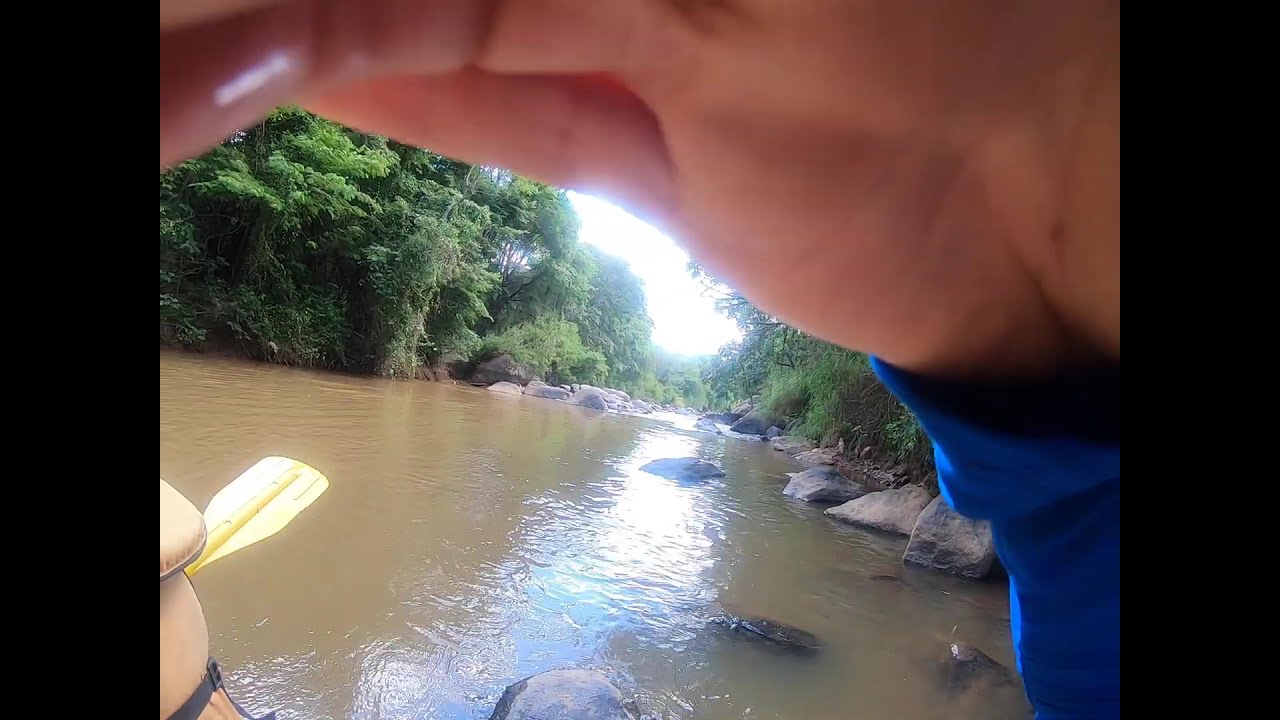A horizontal rectangular image captures a serene yet somewhat mysterious creek scene, bordered by dense trees and brush under a bright, partly cloudy sky. Central to the image is a green, pole-like object, possibly a table leg or something enveloped in seaweed, reflecting a sharp gleam from the sunlight. Below this green structure, the creek showcases varying hues of brown, clearer water in the foreground, and murkier depths behind, accentuated by visible rocky bed formations. In the bottom left corner, a person's hand holding a flat object, adorned with a watch, appears, hinting at activity. Their blue long-sleeved shirt provides a splash of color against the natural setting. They seem engaged in maneuvering an oar, part of which, yellow in color, can be seen at the edge of the photograph. The overall palette of greens, browns, and blues ties together the tranquil yet dynamic tableau of a day spent paddling through this calm, rocky creek.